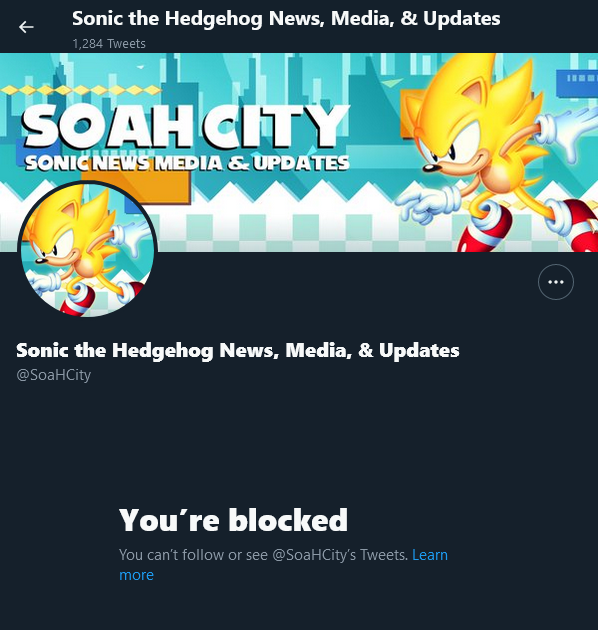The image is a square screenshot featuring a prominent jet black background at both the top and bottom. A black horizontal banner runs along the top, displaying the bold white text "Sonic the Hedgehog News, Media and Updates." Near the upper left-hand corner, a white arrow points to the left.

Dominating the center of the image is an illustration of Sonic the Hedgehog, but with a twist—he is yellow instead of his usual blue. Sonic, clad in his signature red shoes and white gloves, appears to be running and is positioned towards the right side of the composition. The background is an abstract representation of a city, labeled as "SOAH City, Sonic News, Media and Updates."

Beneath this, within a circle, the same image of the yellow Sonic is repeated. Below this circular illustration, more bold white text states, "Sonic the Hedgehog News, Media and Updates," followed by "At SOAH City" in a smaller font.

The lower part of the image features larger bold white text that declares, "You're Blocked." Directly beneath, in smaller white text, it reads, "You can't follow or see @SOAHCity's tweets." A clickable blue link at the bottom says "Learn More," directing users to further details about the block.